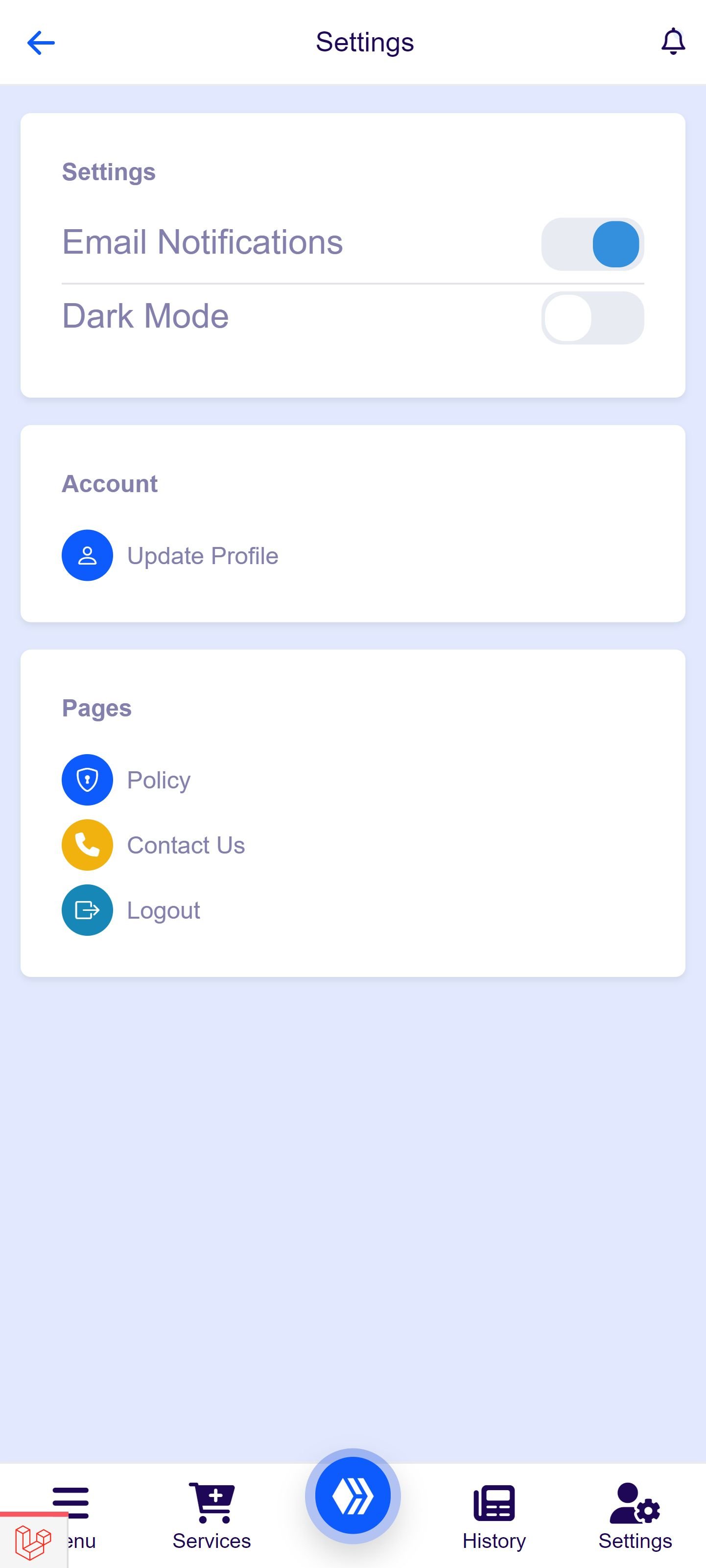This image is a detailed screenshot of the settings tab within a mobile application. The brand name or specific application is not identifiable in the screenshot, rendering it quite generic. The entire image is occupied by the phone screen displaying the settings interface, and no external elements like Wi-Fi bars are visible.

In the upper left-hand corner of the screen, there is a blue back arrow. Centered at the top is the word "Settings," and on the upper right-hand side, there is a small bell notification icon. Below this header, the settings section is reiterated with similar text "Settings." The first option listed is "Email Notifications," which is turned on, followed by "Dark Mode,” which is turned off.

Beneath these settings, there's an “Account” section featuring an option to "Update Profile," accompanied by a blue icon of a person. Following this, there is a "Page" section comprising three options: "Policy," "Contact Us," and "Log Out." Each option is paired with a colored icon: a blue shield-like design for "Policy," a yellow phone for "Contact Us," and a teal door-like icon for "Log Out."

At the very bottom, four tabs are visible for navigation within the application: "Menu," "Services," "History," and "Settings." The "Menu" tab is symbolized by three lines, “Services” by a checkout drawing, “History” by a fax machine icon, and "Settings" by a person with a gear. Centered within the tabs is a distinctive blue circular button featuring three diamond shapes, whose function is unclear. Additionally, in the bottom left-hand corner, there is an ambiguous red and white logo.

Overall, the screenshot captures a detailed, comprehensive view of the app's settings tab, though the app's specific identity remains unknown.